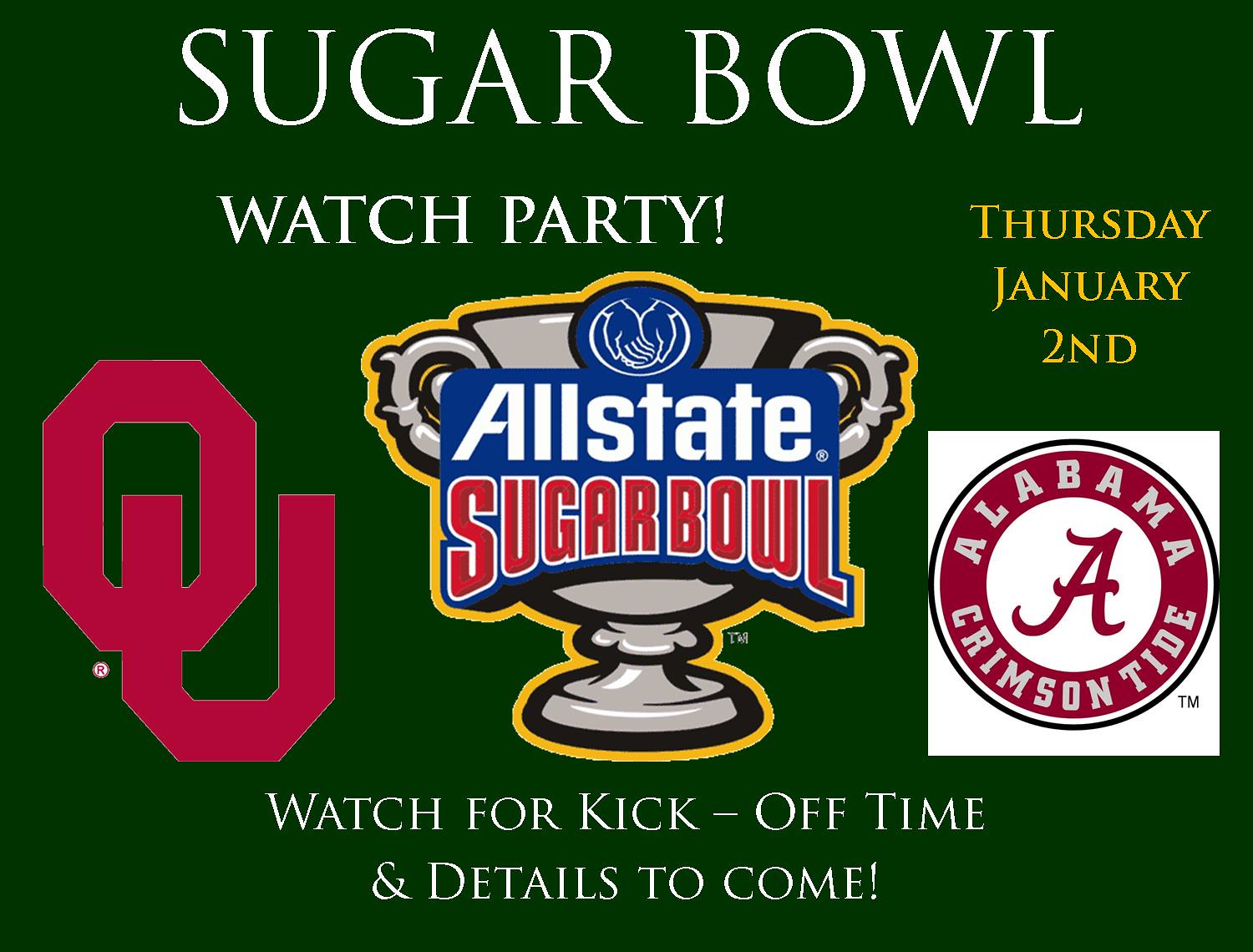The image is a dark green rectangular advertisement for a Sugar Bowl watch party, featuring prominently in white text "Sugar Bowl Watch Party" and "Allstate Sugar Bowl." The "Allstate Sugar Bowl" logo has "Allstate" in white letters and "Sugar Bowl" in red letters on a blue background. Central to the image is a silver trophy cup with a circle above it displaying a picture of two hands. To the left side, the red "OU" logo is visible. The image also includes the text "Thursday, January 2nd" in yellow, alongside "Alabama Crimson Tide" with a large letter "A" in a white circle. At the bottom, in white text, it states "Watch for kickoff time and details to come."